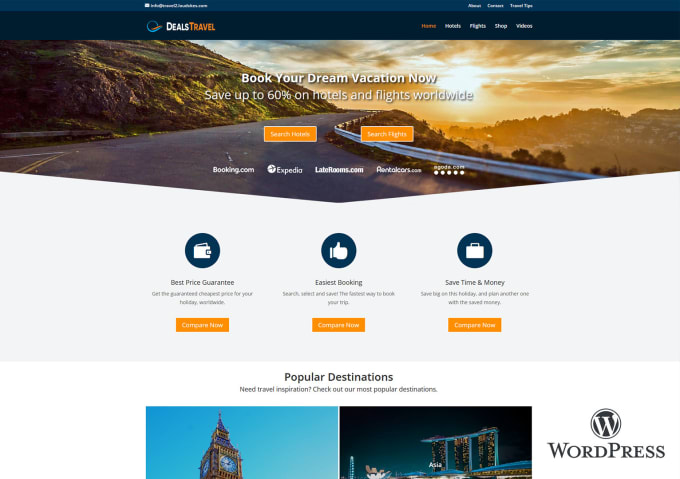The image appears to be a promotional webpage for travel deals. At the top of the page, there is a blue banner with white text that is illegible due to its small size and blurriness. Below it is a darker blue banner featuring a green circle with an orange streak, located towards the right-hand side. The words "deals" and "travel" are positioned closely together, almost forming a single term; "deals" is written in white, while "travel" is in orange. 

Continuing down the page, there are several headings that are also blurry, making them difficult to read, but it appears they may include terms like "flights" and possibly "stop." Beneath these headings is a scenic image depicting a roadway winding around mountainous terrain, with a silver barrier along the road. Superimposed on this image is the text, "Book your dream vacation now. Save up to 60% on hotels and flights worldwide."

The page also features two prominent orange buttons labeled "Search Hotels" and "Search Flights." Below these buttons are logos of various travel service providers such as booking.com, Expedia, Lotsofrooms.com, and an additional, unreadable logo. The overall aesthetic and content suggest that this page is designed to entice users to explore and book travel deals.